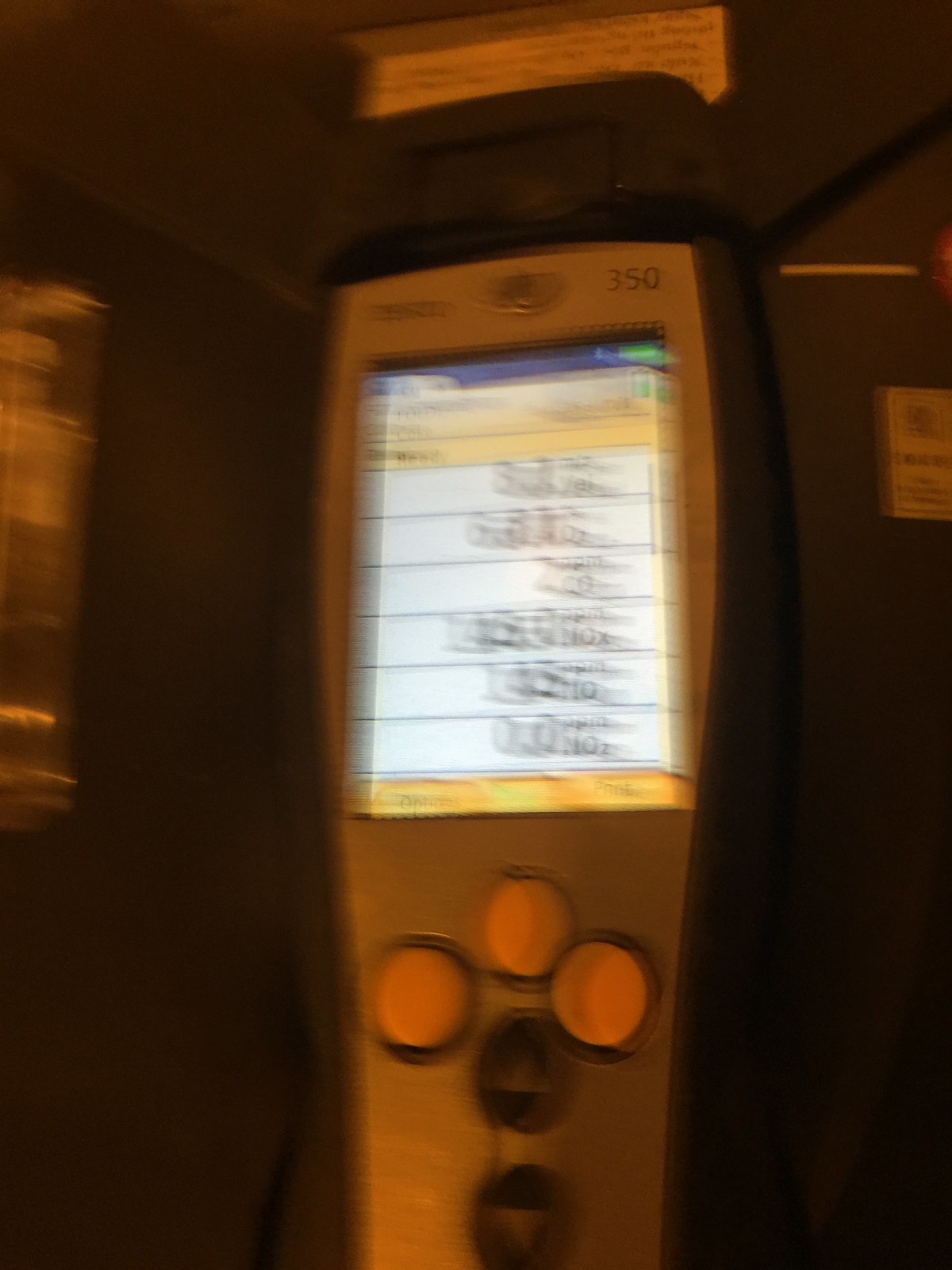This image features a very blurry close-up of a digital remote control, exhibiting a somewhat confusing design and surrounding elements. The remote has a white screen display on the top half. The screen has dark blue, green, yellow, and white colors, with blurred black text that is unreadable. Below the display, there are three round orange buttons used to unlock the remote, followed by two black buttons with up and down arrows for navigation. The remote control is predominantly silver-gray in the middle, encased in black plastic that is curved in the center and flares out towards the bottom, giving it a rounded rectangular shape. There appear to be additional buttons or markings on the device, possibly representing rows of measurements, but they are indistinct due to the blurriness. The entire scene has a gray or black surroundings, with reflections suggesting strong indoor lighting, and hints of a red hue, perhaps indicating a nighttime or enclosed setting.